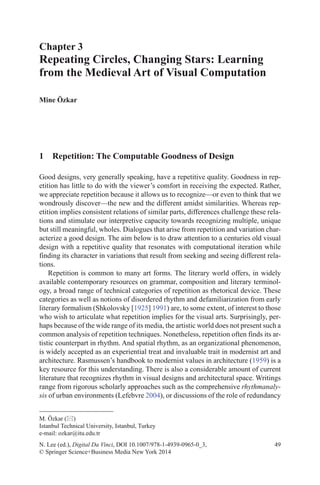The image depicts a page from a book or possibly a digital excerpt of one, showcasing predominantly black text on a white background. At the very top, it specifies "Chapter 3," followed by the chapter title, "Repeating Circles, Changing Stars: Learning from the Medieval Art of Visual Computation." Beneath the title, the author's name is indicated, presumed to be Mein Oskar, affiliated with Istanbul Technical University, Istanbul, Turkey, and providing an email address. The page features a section title, "1. Repetition: The Computable Goodness of Design," followed by two paragraphs of textual content that elaborate on design principles, which are not fully legible. At the very bottom, there are references listed, presumably citing sources related to the discussed topics.